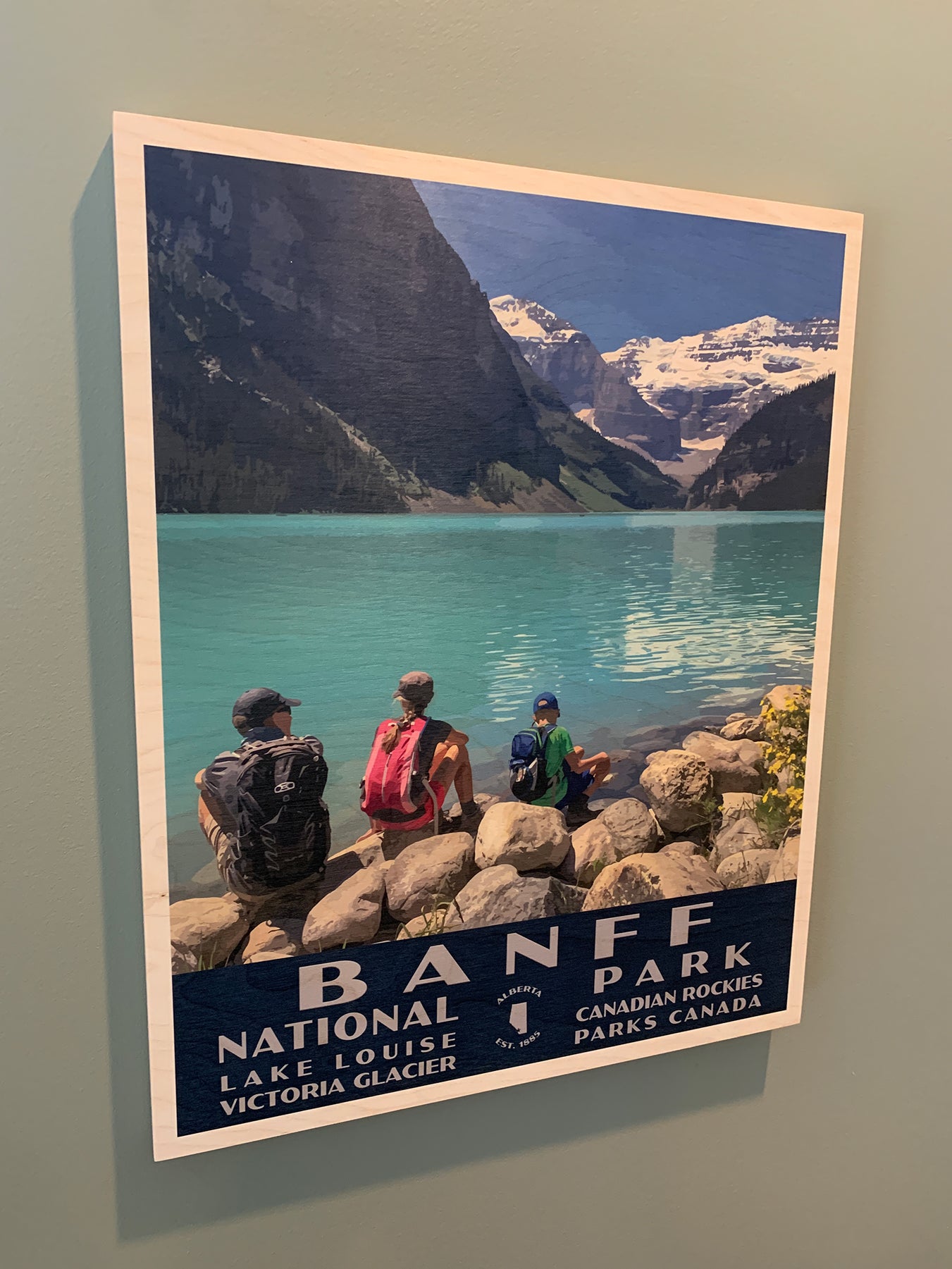The image depicts a poster hanging on a greenish-gray wall. The poster, framed by a light tan border, showcases a stunning landscape of Banff National Park in Canada. It features vibrant turquoise waters of Lake Louise, surrounded by a mixture of dark gray and snow-capped mountains. A clear blue sky peeks through in the upper right corner. In the foreground, three individuals—each donning t-shirts, baseball caps, and backpacks—sit on large gray rocks, gazing at the lake. The person on the left wears blue with a matching backpack, the one in the middle sports a dark shirt with a red backpack, while the person on the right is dressed in green with a blue backpack. Moss is visible on the right side of the rocks. At the base of the poster, white text reads: "BANFF National Park, Lake Louise, Victoria Glacier, Canadian Rockies, Parks Canada."